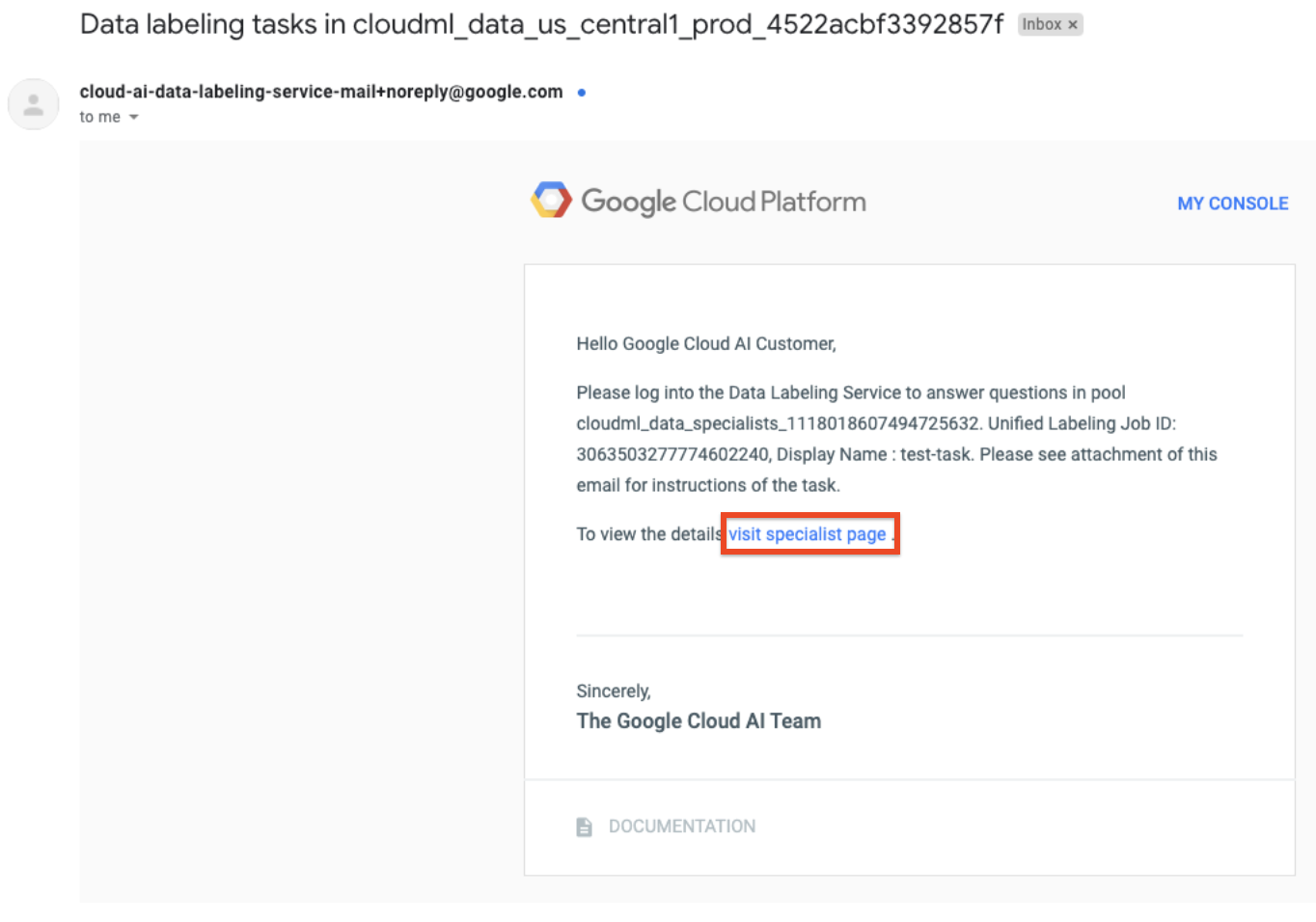**Screenshot of Received Email Detailing Data Labeling Tasks in Google Cloud ML Platform**

The image presented depicts a screenshot of an email received from Google's AI Data Labeling Service. The email subject is prominently titled: "Data Labeling Tasks in Cloud ML_US_Central1_Prod_4522ACPF3392857F". Above the email content, a small grey box labeled "Inbox" is visible.

The sender information on the left-hand side lists "Cloud AI Data Labeling Service" with the sender email "mail+noreply@google.com". Below this, the email is addressed "To: Me", indicating it was directed to the recipient's inbox.

The main body of the email is shown in the center of the image, with the header "Google Cloud Platform". The email greets the recipient as "Google Cloud AI Customer" and continues with a request: "Please log into the Data Labeling Service to answer questions in pool, Unified Labeling Job ID: Display Name Test Task". The email instructs the recipient to check the attachment for detailed instructions related to the task and to visit the specialist page for further information.

The final part of the message, which provides a navigation link, is highlighted in blue and bordered by a red box, visually distinguishing it from the rest of the content.

Overall, this screenshot provides a comprehensive and instructive look at an email template used by Google Cloud's AI Data Labeling Service to inform users of new tasks and necessary actions.